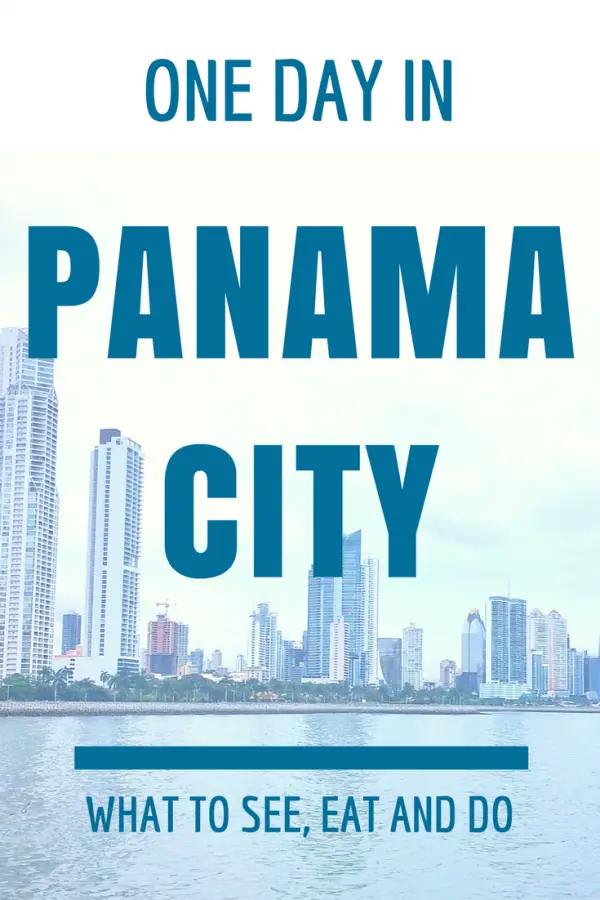The image is a promotional webpage for "One Day In." At the top, the title "One Day In" is prominently displayed in blue. The background features a picturesque scene of Panama City, showcasing a skyline of tall skyscrapers that gradually decrease in height from left to right. The tallest building is positioned on the far left. In addition to the skyscrapers, there are visible palm trees, a beach, and a body of water, likely the ocean, contributing to the scenic coastal atmosphere.

Beneath the scenic panorama, a horizontal dark blue bar spans the width of the image. In the foreground, centrally positioned, the words "Panama City" are overlaid in dark blue, bold letters atop the skyscrapers' image. Just below this, in smaller, clear text, the words "what to see, eat, and do" guide viewers on activities in Panama City. The upper part of the background consists of a sky filled with predominantly white clouds, enhancing the overall airy and inviting feel of the webpage. This visual composition effectively conveys a day-trip guide to Panama City, emphasizing key attractions and activities.